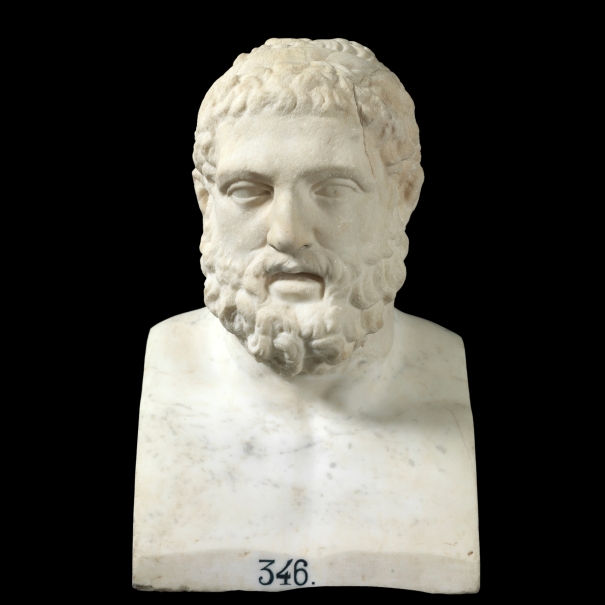The image depicts a striking bust of a man from ancient times, sculpted from a marbled white stone with gray streaks. The man has short, curly hair and a short, textured curly beard, complemented by a mustache. His intense stare is accentuated by white eyes featuring small gray dots in the center. The bust is mounted on a large square base that also exhibits the marbled white and gray pattern. This base prominently features the number "346." The sculpture stands out dramatically against a solid black background, emphasizing its fine craftsmanship and the detailed features of the bust.